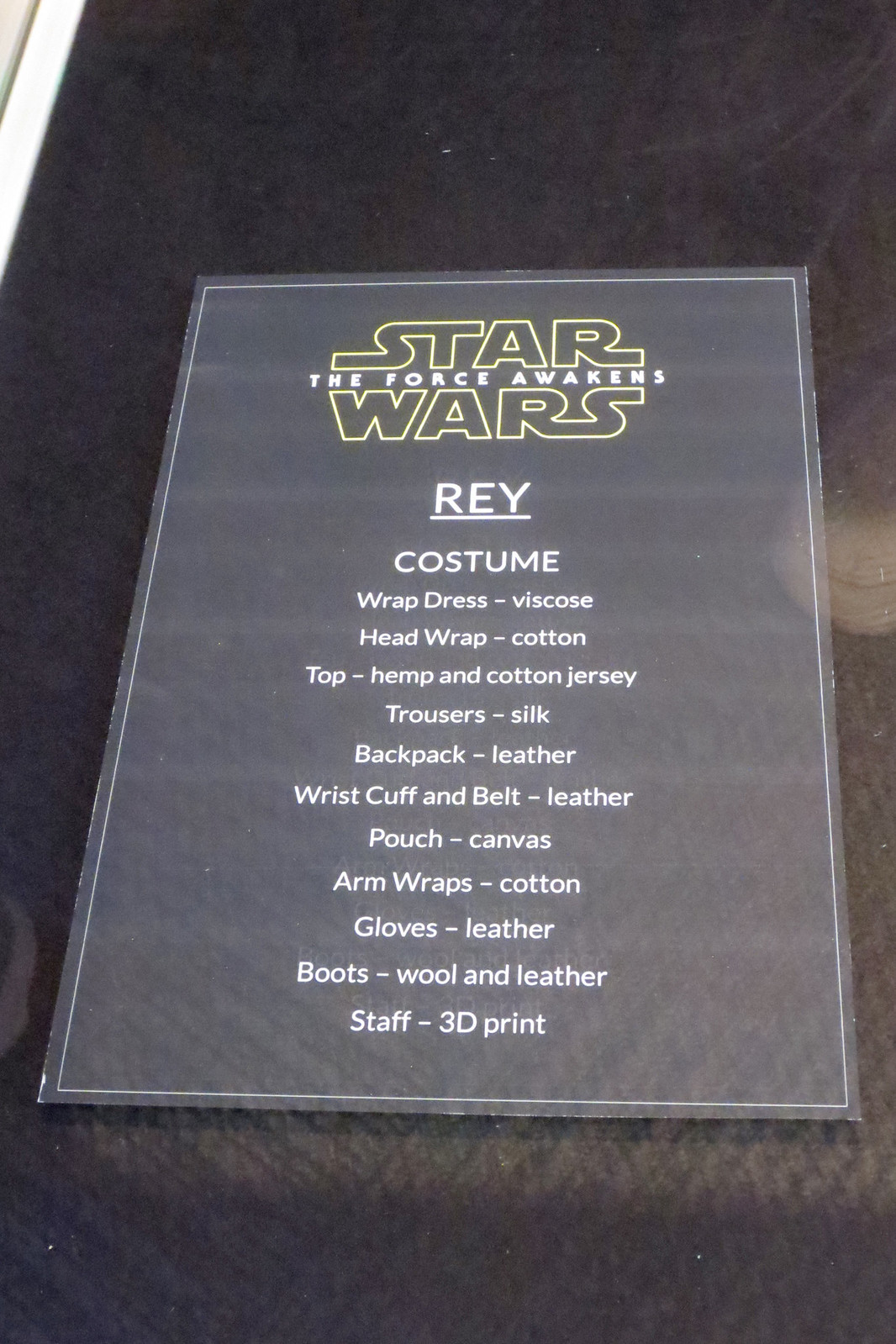Set against a black fabric background, the image features a centrally placed informational card describing the costume of Rey, a character from Star Wars: The Force Awakens. The black rectangular card, bordered in white, has the iconic Star Wars logo at the top, followed by "The Force Awakens" in white text. Below this, the card details the components of Rey's outfit: a viscose wrap dress, a cotton head wrap, a hemp and cotton jersey top, silk trousers, a leather backpack, leather wrist cuff and belt, a canvas pouch, cotton arm wraps, leather gloves, and boots made of wool and leather. Additionally, it notes that Rey's staff is a 3D print. This descriptive card, reminiscent of an exhibit display, suggests it might be part of a Star Wars memorabilia exhibition, perhaps within a costume store, and is placed on an indeterminate dark material that highlights its content. The prominent colors in the image include black, white, gray, yellow, and tan.